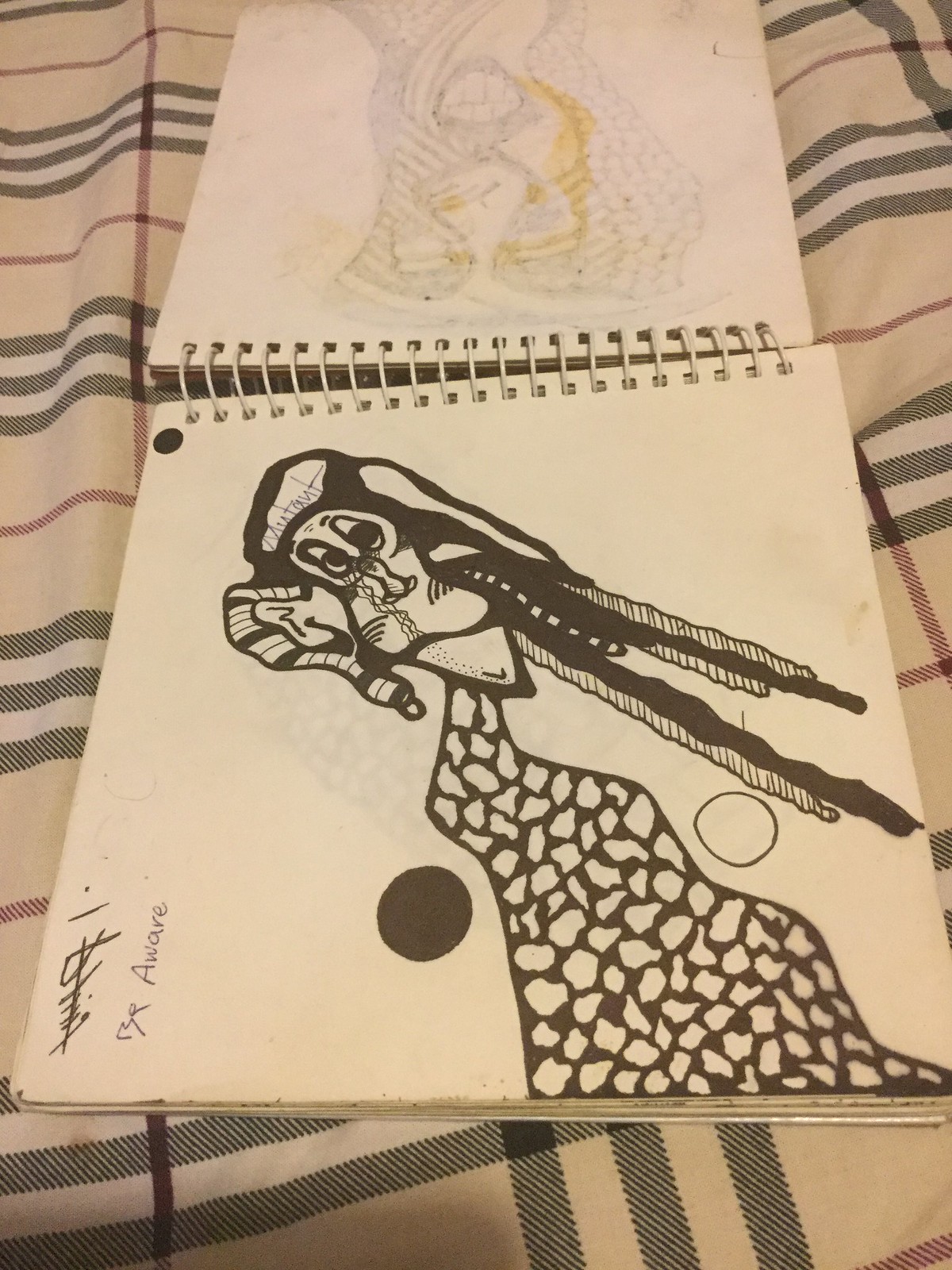This photograph captures an open, spiral-bound sketchbook placed on a beige plaid sheet, resembling a Burberry pattern with black, white, and rust-colored lines intersecting. The sketchbook shows signs of wear, suggesting frequent use. The visible page features a striking black and white drawing of a cartoonish figure with a human body dressed in a long black gown adorned with irregular white spots. The figure has distinctive dreadlocks, with some sections covered by patterned scarves or headpieces, extending almost to its knees. The face is peculiar, including a duck-like nose and triangular mouth, with one human-like ear wrapped in cloth. Above the character, there are two circles—one black and one white. The background page shows marker bleed-through from prior artwork. In the bottom left corner of the drawing, the words "be aware" are carefully inscribed in pencil.